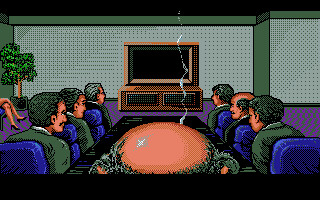In this pixelated, old-timey video game scene, we see a detailed depiction of a conference room viewed from behind a bald man seated at the head of a rectangular table. The man's bald head glistens under the light, with tufts of hair on the sides and smoke rising from a cigar in front of him. The conference table, flanked by six men in green suits with white shirts, is black, and the occupants are seated on blue chairs. The men's hair varies from dark to gray, with one additional bald individual among them.

The focal point of the room is an antique, wood-encased television set with a distinctly large, protruding back, reminiscent of monitors from the 80s. This TV, which has two small black cabinets underneath, draws the attention of everyone in the room. Surrounding the table is a purple carpet, while the walls are painted in varying shades of green, and the ceiling is black. There's a pink item emitting an aroma on the table, hinting at food or another scented object.

On the left side of the image, we glimpse a pair of women's legs in black pumps, possibly belonging to a note-taker, sitting next to a potted plant. The digital graphic style, with a black border banner on both the top and bottom of the image, adds a whimsical, animated touch to the overall scene.